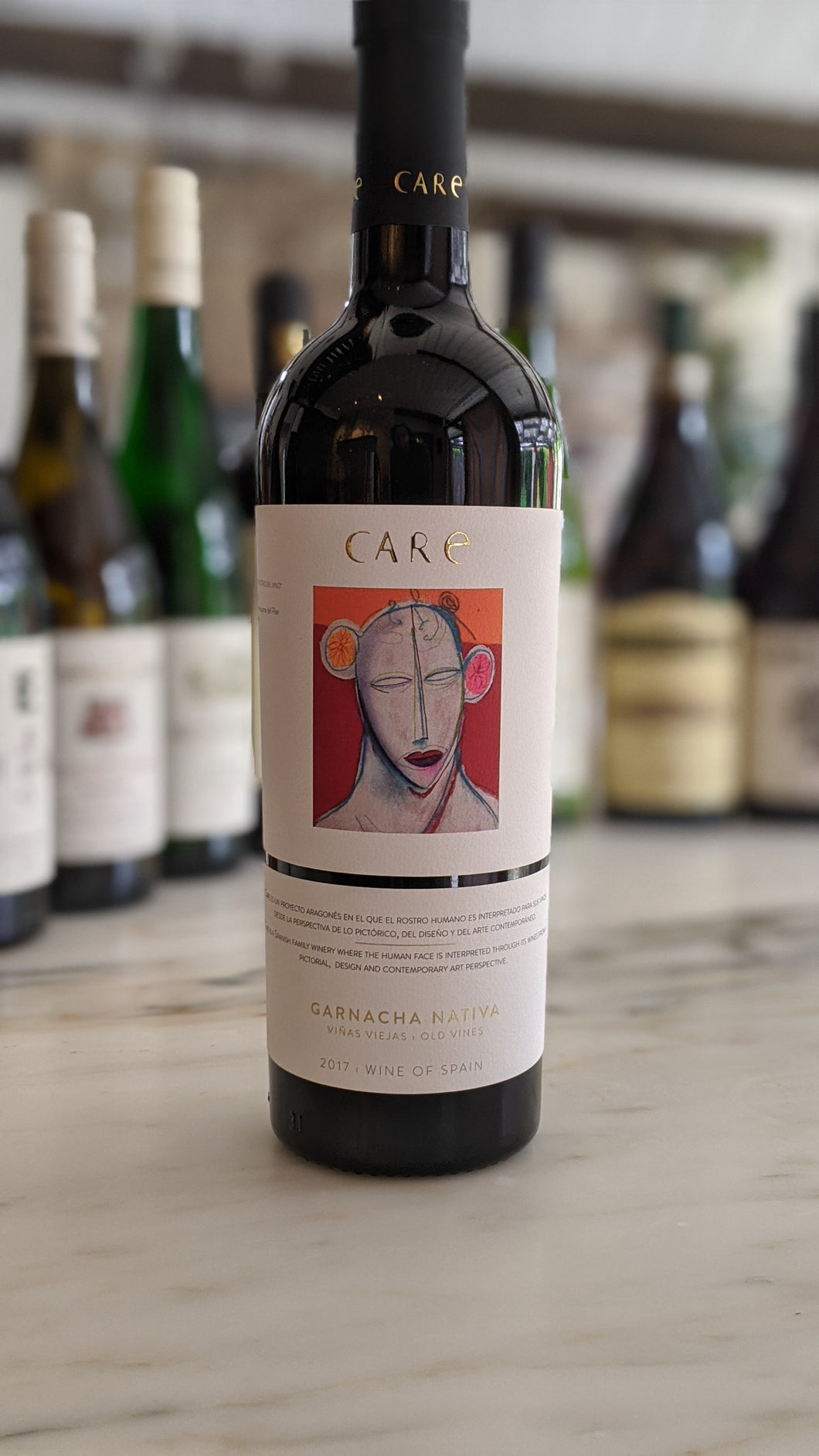This photograph captures a striking bottle of wine prominently positioned at the center of the composition. The featured bottle, with an almost black hue, stands on a white and gray table. In the background, there are seven other wine bottles that are deliberately blurred to highlight the centerpiece.

The label on the wine bottle is tan and showcases a unique piece of artwork. This artwork depicts a stylized figure with distinct features: white with red lips, a narrow nose that extends upward through the forehead, and off-center, monkey-like ears. The figure appears to be female with an oval-shaped face and a thick neck.

The name of the wine, "C-A-R-E," is printed above the image on the label. Additionally, the name "C-A-R-E" is embossed in gold on the bottle's neck, adding an element of elegance. This bottle of wine remains unopened, preserving its pristine appearance. The overall setup, with the in-focus bottle set against the slightly out-of-focus background bottles, creates a sophisticated visual depth.